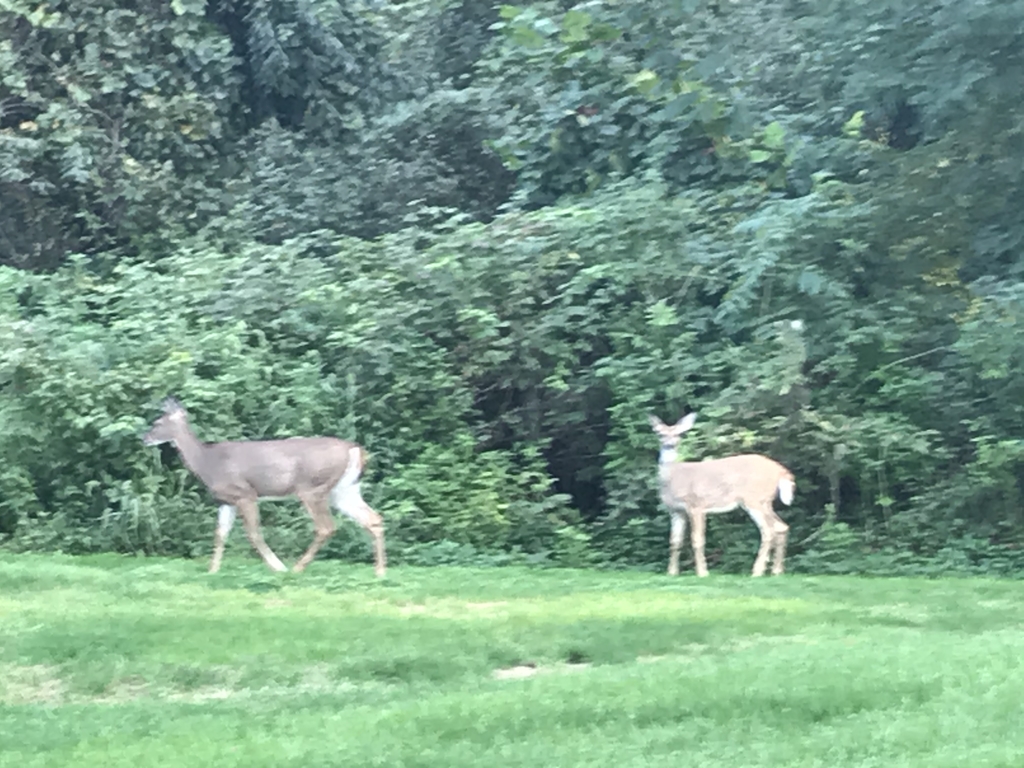In this daytime image, two deer stand in a vibrant, green yard bordered by dense woods. The foreground features an overgrown grassy field, rich with patches of lighter and darker greens, suggesting a natural, unmowed environment. One deer, a darker brown, stands on the right, while a lighter beige deer, likely younger, with a white tail looks directly at the camera in the center of the field. The scene appears subtly blurred, indicative of a motion shot. The background is densely packed with various trees, leaves, vines, and shrubs, creating a lush forest edge. The season is likely spring or summer, given the bright, healthy foliage and vivid natural colors. The deer, both without visible horns, are medium-sized and central to the composition, adding a serene wildlife aspect to the picturesque setting.